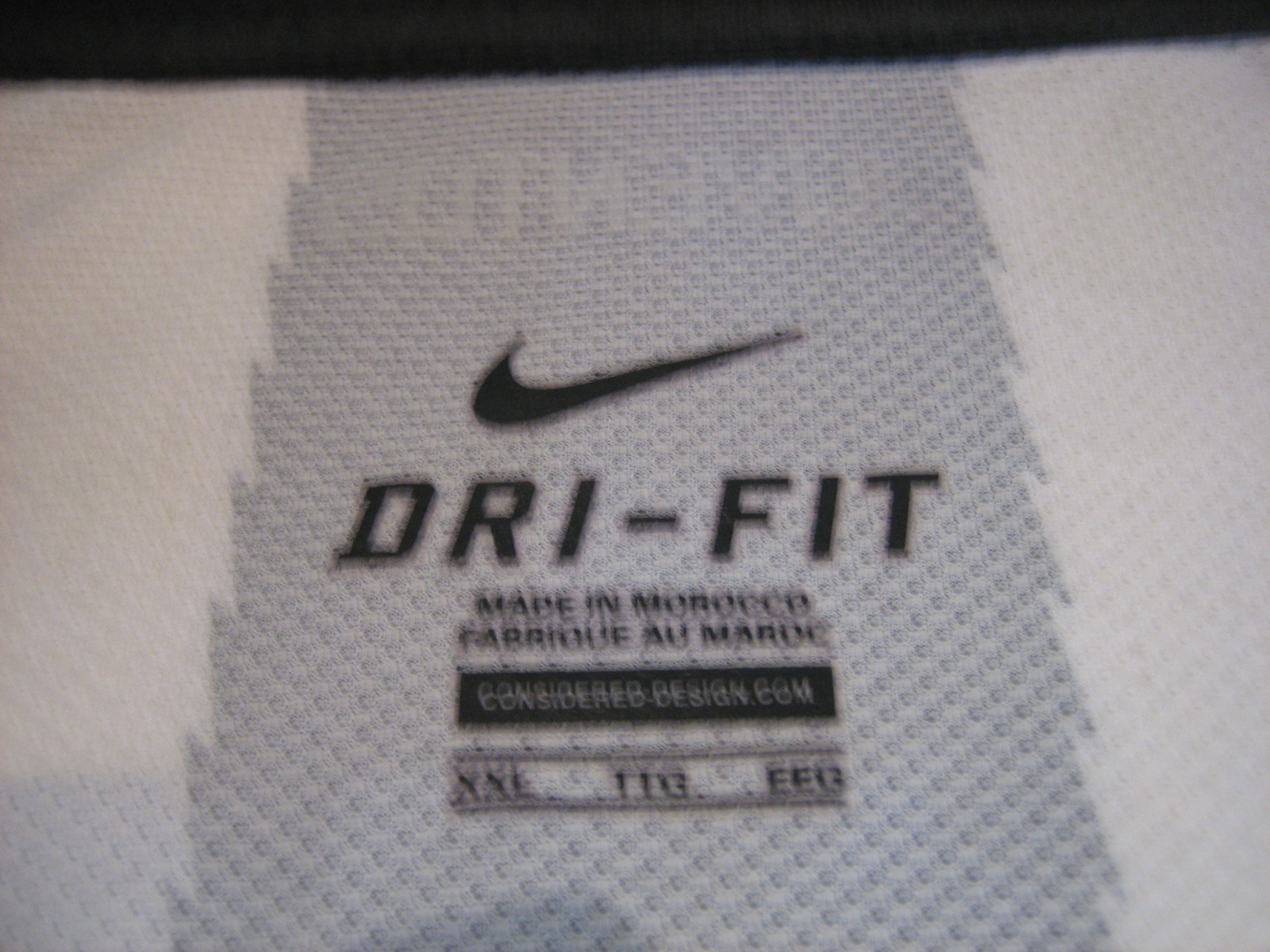The image depicts a slightly blurry, close-up shot of a label inside a Nike Dry-Fit clothing item. The fabric showcases a textured, mesh-like honeycomb pattern, predominantly white with a central gray strip visible beneath a black zig-zagged stripe that appears to bleed through from the other side. The label prominently features the iconic black Nike swoosh logo, positioned above the text "Dri-Fit" in black letters. Below this, the tag reads "Made in Morocco" and "Fabriqué au Maroc," followed by the website "ConsideredDesign.com." The size of the garment is listed as XXL (also shown as TTG and EEG). The overall image only captures about four to five inches of the fabric, which is crafted from typical athletic material consistent with Nike's Dry-Fit line.